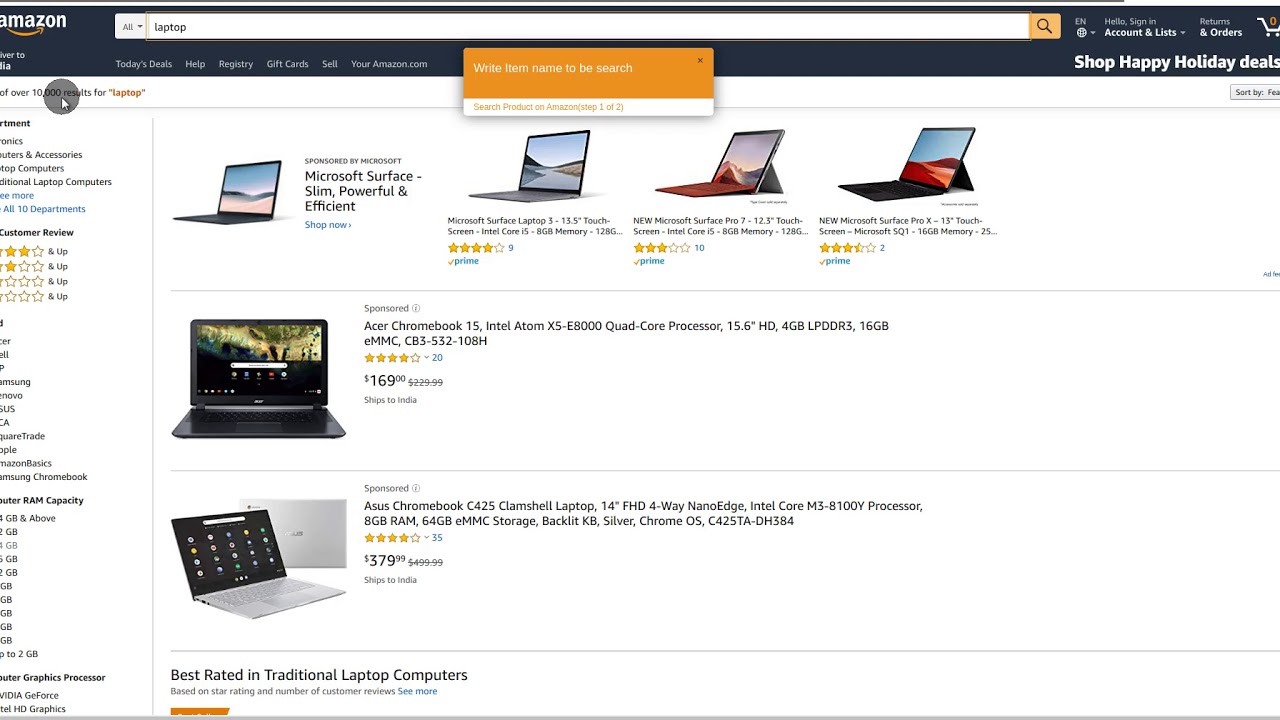This screenshot captures a user browsing for laptops on Amazon. The familiar Amazon logo is prominently displayed in the top left corner, and the top navigation bar is black with orange accents. The search bar is set to search within all departments and currently has "laptop" entered as the search term. An orange magnifying glass icon, used to initiate the search, is visible on the right edge of the search bar.

In the top right corner of the screen, the user's account options are displayed, including "Hello, Sign in," "Account & Lists," the language selection set to English, "Returns," "Orders," and a shopping cart icon showing zero items. Below the main navigation bar, a banner reads "Shop happy holiday deals."

A semi-transparent orange pop-up appears, prompting the user with "Write item name to view search" and "Search product on Amazon, Step 1 of 2." The search results for "laptop" are prominently displayed, featuring multiple laptops. Each laptop is shown facing to the left with open screens. 

Two laptops are highlighted vertically: the "Acer Chromebook 15" and the "Asus Chromebook C425." Below this, a section labeled "Best rated in traditional laptop computers" is visible. On the left side of the screen, partial filtering options can be seen, including categories like "Department" and "Customer Reviews." The bottom part of the screenshot is cut off, so not all filtering options are visible.